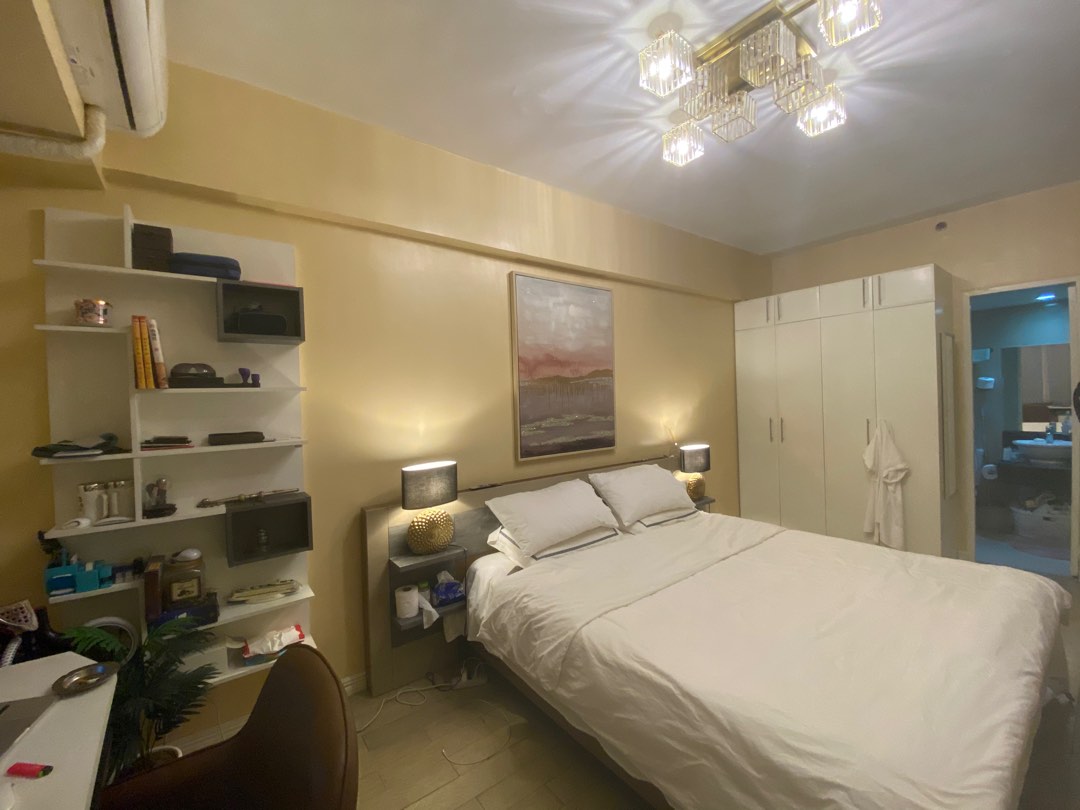In this image, the ceiling is painted white and features a central gold light fixture. The ceiling is accented by four individual light fixtures arranged in a square, creating a white outline. The back wall is painted yellow, adorned with a square picture that showcases a painting in shades of orange and gray. Positioned centrally is a bed made up with off-white bed sheets and two off-white pillows.

Flanking either side of the bed are gray rounded light fixtures with gold bowls shadowing the light sources. These fixtures sit atop short, gray shelving units that have a gray background. One of these units holds a roll of toilet paper and a blue tissue box.

On the right side of the room, there's a white, square clothing cabinet. A white shirt is hanging on one of the door handles. Adjacent to the cabinet, there is a white door frame leading into another room illuminated by a soft blue light.

To the left side of the room, a white shelving unit boasts a variety of objects: black screens at the top, brown books on the upper shelves, and silver rounded jars on the lower shelves. The floor is a light brown color, complementing the room's overall aesthetic. Also on the left is a white table accompanied by a brown chair with a rounded back.